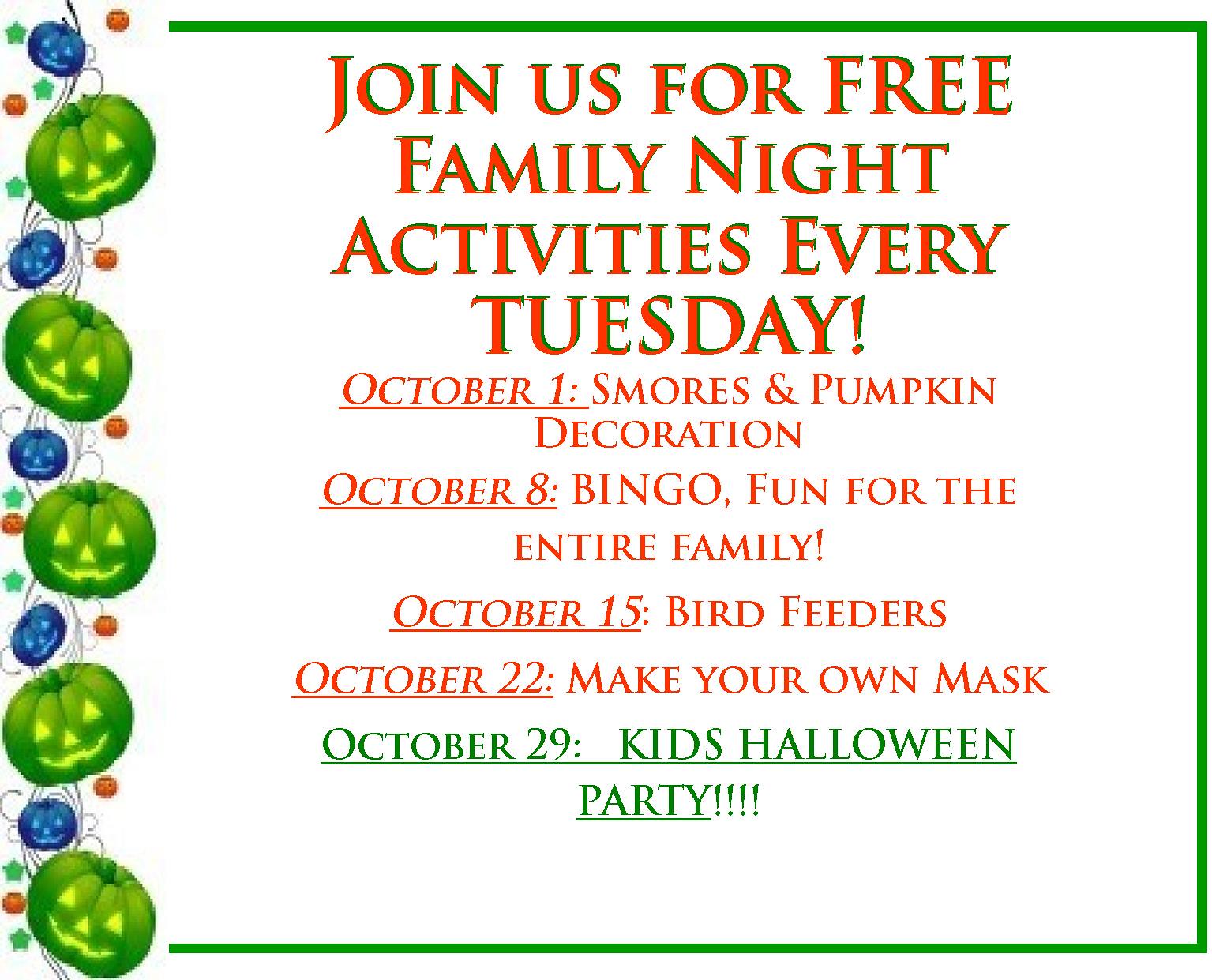This digital event invitation features a vibrant and festive design perfect for October. Dominating the left side of the image is a vertical line of alternating blue and green jack-o'-lantern-shaped pumpkins. The blue pumpkins, smaller and tilted to the right, alternate with the larger green pumpkins that tilt to the left. Interestingly, this pattern changes briefly as two pumpkins in the middle sit flat before resuming their alternating tilts. Enclosing the entire design is a green border on three sides: the top, right, and bottom. The central background of the invitation is red with the event text prominently displayed in red font with a green outline. 

It reads: "Join us for free family night activities every Tuesday" and lists the following events: 
- October 1st: S'mores and pumpkin decorations
- October 8th: Bingo! Fun for the entire family
- October 15th: Bird feeders
- October 22nd: Make-your-own-mask 

In bold, capitalized green text, it further announces the highlight: 
- October 29th: KIDS HALLOWEEN PARTY. 

This carefully designed invitation merges playful holiday-themed imagery with comprehensive event details, perfect for bringing families together in October for a series of exciting activities.